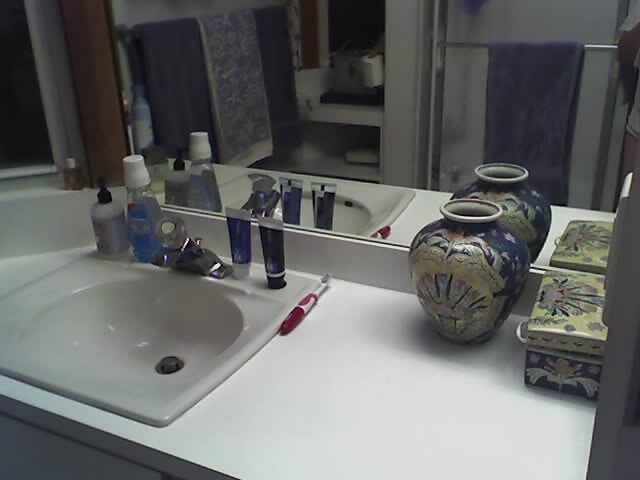A well-lit bathroom featuring a pristine white sink occupies the center of the photo. To the left of the sink, there's a bottle of mouthwash, essential for maintaining oral hygiene. A tastefully arranged vase graces the countertop, adding a touch of elegance to the space. On the right side, a chest serves as additional storage. In the foreground, a toothbrush is positioned on the countertop, accompanied by two containers of gel, likely used for hairstyling. The overall scene is a clean and functional bathroom setup with thoughtful details that blend utility and aesthetics.